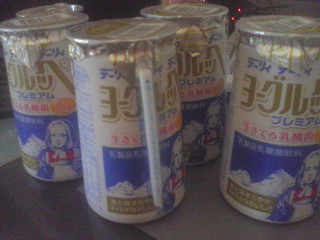The image depicts a close-up view of four cylindrical cans of a beverage, each with a detailed and distinct label. The cans feature a white background adorned with golden and blue lettering in a foreign language. At the bottom of each can, a rectangular picture showcases a blue sky, snow-capped mountains, and an illustration of a European girl dressed in a blue bonnet, red shirt, and white pinafore. These cans are topped with a square piece of silver foil, its corners hanging over the edges, and a white straw attached to the side of each can. The cans are placed on a flat surface that transitions from dark brown to light gray. The background includes a slightly visible dark upper section with two small, glowing red or orange lights in the top right corner, adding a touch of mystery to the setting.